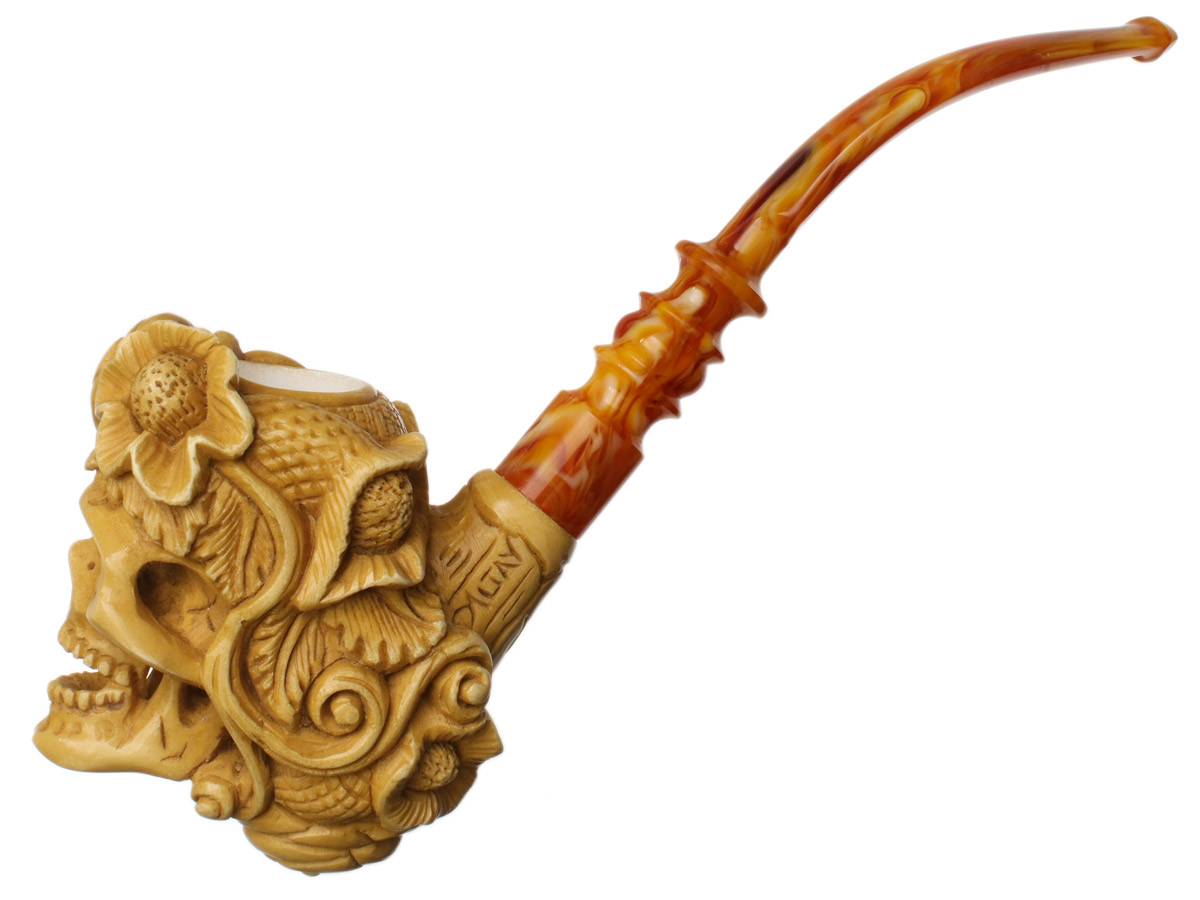The image features an ornate, vintage-style smoking pipe set against a stark white background. The pipe stretches diagonally from the lower left corner to the upper right corner. It is crafted from a glossy material with intricate wavy lines in shades of brown, orange, and white, resembling marble. The stem of the pipe is curved and detailed with inlay grooves, enhancing its elegant design. The bowl, which is situated at the base of the stem, appears to be made from a bone-like material with a yellowish tint, giving it an antiquated feel. 

The most striking feature of the pipe is the intricately carved skull adorning the front portion. The skull faces the lower left corner, with its mouth open, showcasing detailed teeth and a prominent jawline. Its hollow eyes are hauntingly set. Atop the skull, an ornate hat featuring a profusion of curly designs, including spirals and leaves, adds to the royal aesthetic. Above the left eye of the skull, a carved flower stands out amidst the intricate patterns. The overall design, with its combination of carved curves, textural details, and royal patterns, makes this pipe a standout piece of craftsmanship.